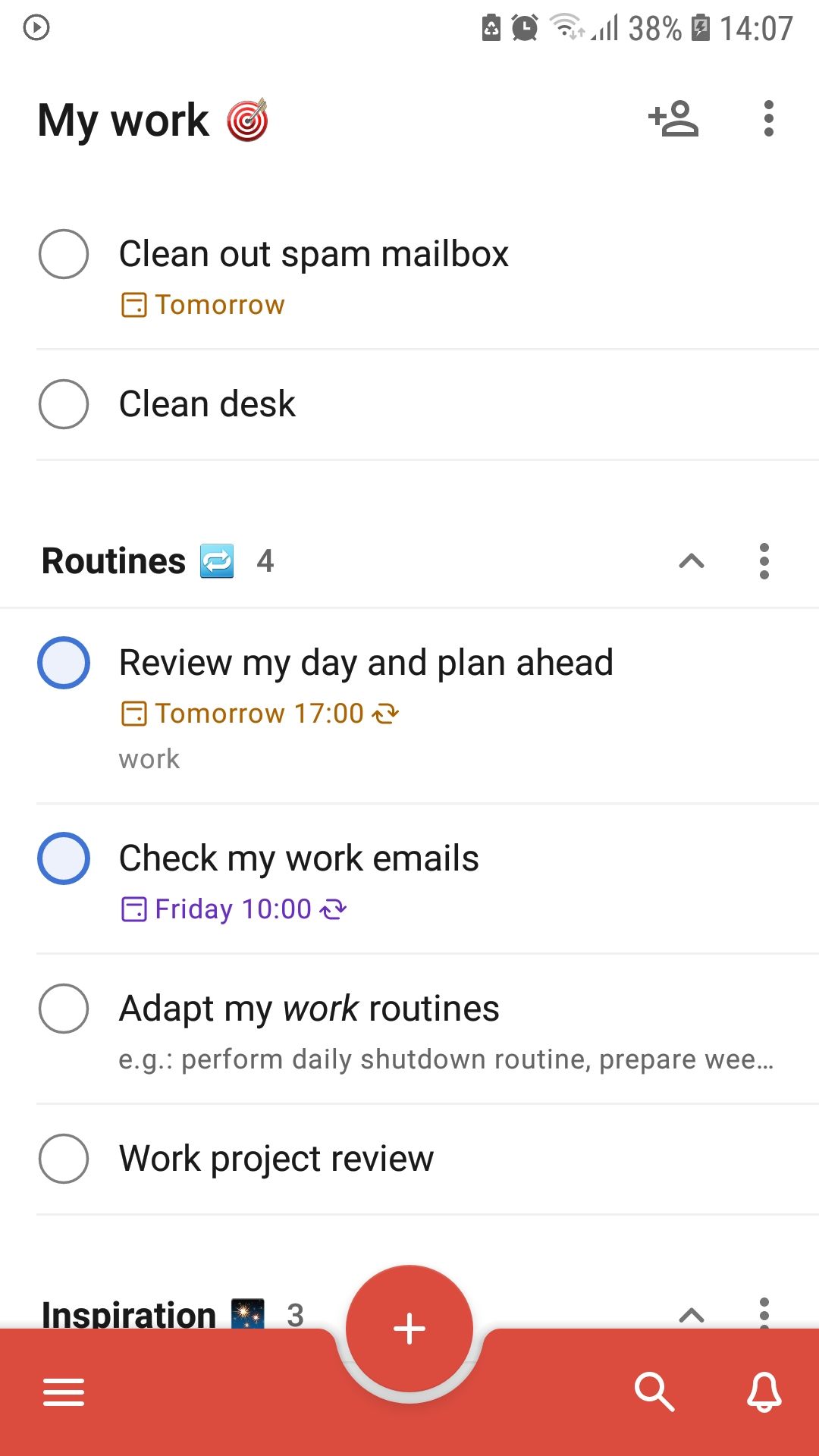This is a detailed screenshot from a to-do list app interface. The image prominently displays three categorized to-do lists against a clean white background, with all text rendered in black for clarity. 

1. **Top To-Do List - My Work (🎯)**
   - Title: **My Work** followed by a bullseye emoticon (🎯)
   - Tasks:
     - **Clean Out**: Identified by a grey circle on the left
     - **Spam Mailbox**: Identified by a grey circle on the left
     - **Clean Desk**: Identified by a grey circle on the left

2. **Middle To-Do List - Routines (🔄)**
   - Title: **Routines** accompanied by a blue cycle icon, representing two arrows feeding into each other (🔄)
   - Tasks:
     - **Review My Day and Plan Ahead**
     - **Check My Work Emails**
     - **Adapt My Work Routines**
   
3. **Bottom To-Do List - Inspiration (🌌)**
   - Title: **Inspiration** with a space-themed emoticon (🌌)
   - Note: The tasks in this list are partially obscured and not fully visible in the screenshot.
   
Below the to-do lists, there's a large horizontal orange rectangle forming a bottom bar. On this bar, from left to right:

- **Hamburger Menu**: Positioned on the far left
- **Add Task Icon**: Represented by a circle with a plus icon in the center
- **Search Icon and Bell Icon**: Aligned to the right side

The overall interface is visually structured and organized, with clear indicators for tasks and interactive elements.